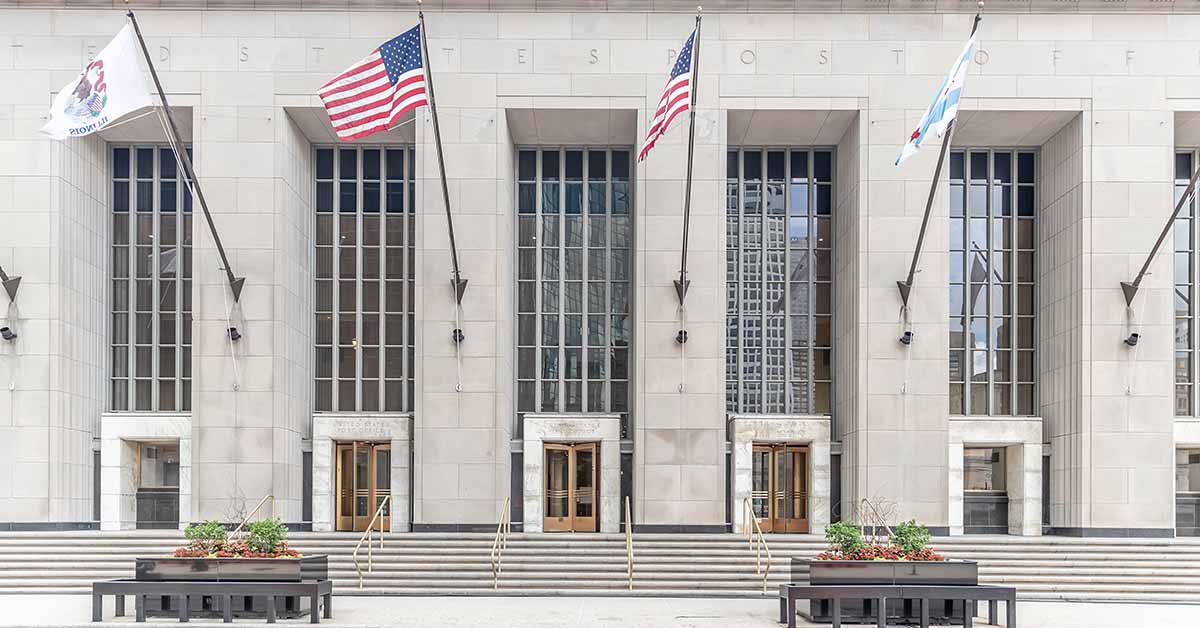This image captures the majesty of a United States Post Office building situated in a bustling metropolis. Dominating the scene is the building's grandiose stone façade, exuding a sense of timeless elegance and strength. The structure features a series of expansive glass windows stretching upward, encompassing three additional stories above the entryway, allowing natural light to flood the interior spaces. 

The entrance is marked by three revolving doors, flanked by supplementary walk-up service windows, serving as portals into this architectural marvel. Intricately designed stone pillars stand as sentinels before the building, each adorned with flagpoles. Proudly waving are two American flags, accompanied by several other flags—likely representing various states or other entities.

Leading up to this impressive entrance are wide stone steps, bordered by beautiful planters that host a collection of well-maintained trees, adding a touch of natural beauty to the urban setting. Benches placed strategically around these planters invite visitors to sit and admire the meticulously maintained surroundings. This post office stands as a testament to civic pride, its stately and meticulously designed exterior reflecting the grandeur and historical significance of the services it houses.